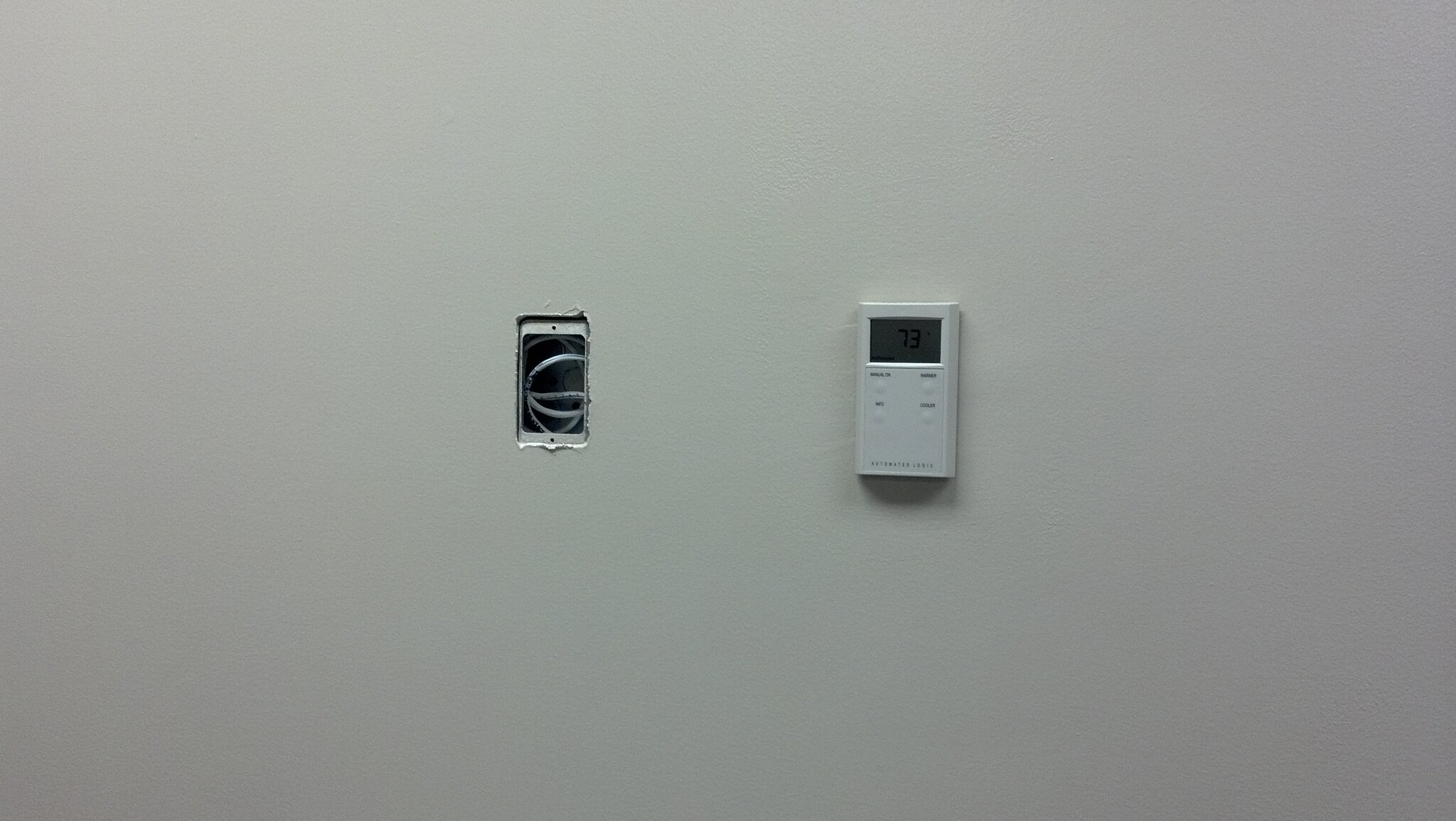In the image, a white wall serves as the backdrop for two primary features: an exposed hole where a light switch or plug might typically be installed, and a digital thermostat. The hole, located slightly to the left of the center, has rough, jagged edges and reveals a rectangular metal plate both at the top and bottom of the cavity. Each metal plate features a central hole designed for securing screws, and visible within this opening are a few wires: two near the top plate, one of which extends just above the center, another slightly below, while a final wire descends to touch the bottom plate.

To the right of this hole, occupying a central position on the wall, is a thermostat slightly larger than the exposed cavity. The thermostat, colored in a yellowish-white hue, prominently displays a digital screen in the upper third showing the temperature set to 73 degrees Fahrenheit in black digits. Below the screen, several raised buttons are interspersed with indiscernible lettering, aligned in a pattern with the first button situated to the right, followed by others sequentially positioned to the left and underneath. Faint lettering runs across the bottom of the unit, though it is not legible in the image. A subtle shadow is cast below the thermostat, adding depth to the depiction.